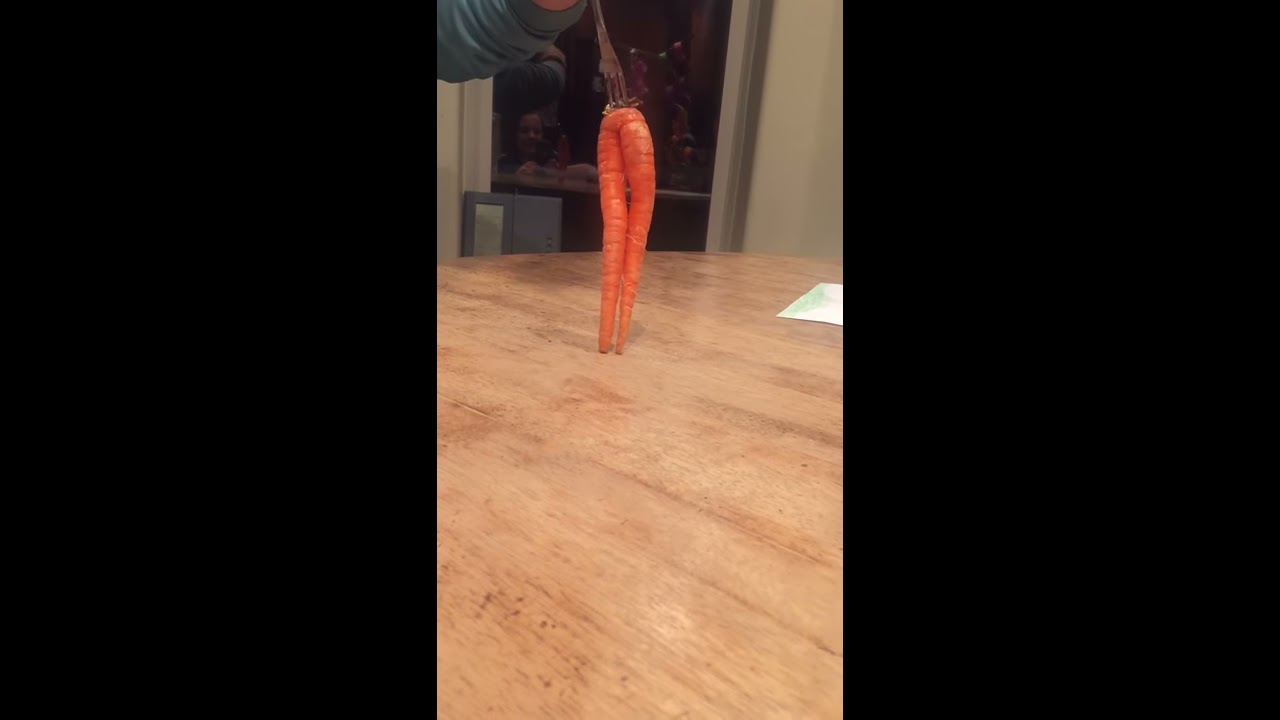The image features a horizontally aligned rectangular frame with solid black side panels on the left and right, and a narrow vertical central area containing the photograph. In the center, there is a light brown woodgrain kitchen table or countertop. Prominently displayed on the table are two connected carrots, positioned such that they resemble human legs. A fork is impaled at the top of these carrots, giving the impression of long legs with the two carrot stems dangling down. The fork is held by an arm dressed in a dark gray long sleeve shirt, with only a bit of the wrist and the spokes of the fork visible. In the background, there is a window, through which the reflection of at least one smiling person can be seen. The window is flanked by white walls, adding further context to the setting. The overall composition evokes an amusing scene, perhaps suggestive of a playful moment where the carrots are imagined to dance with the aid of the fork.